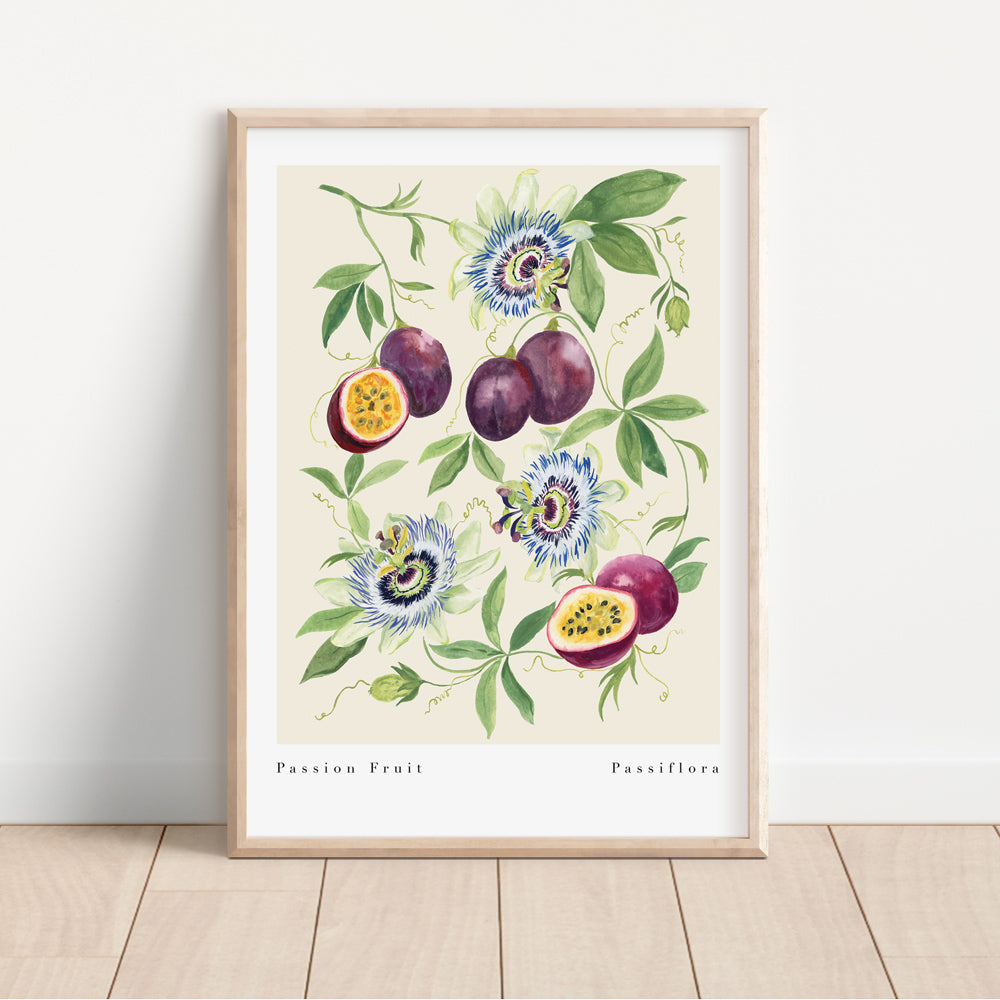The image showcases a photorealistic watercolor painting of six purple passion fruits, two of which are sliced open to reveal their yellow interiors filled with black seeds. Accompanying the fruits are blue passion flowers with intricate white and deeper blue centers, interspersed with green leaves and delicate vines. The painting is housed in a light brown wooden frame with a white matting, and beneath the artwork, small text reads "passion fruit" on one side and "passiflora" on the other. The frame leans against a stark white wall and rests on a light wooden floor. Overall, the layout and naturalistic details capture the essence of the passion fruit plant beautifully.